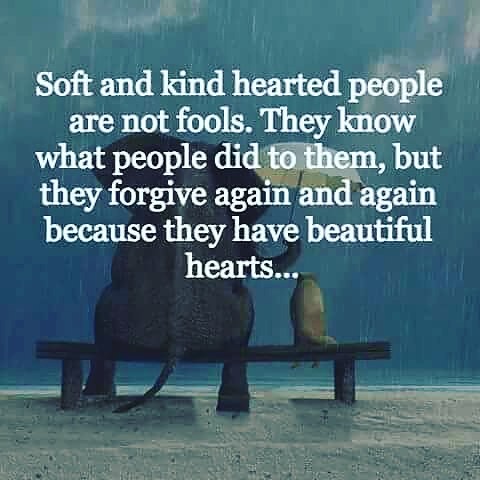The image showcases a motivational poster with an inspirational quote in white text that reads: "Soft and kind-hearted people are not fools. They know what people did to them, but they forgive again and again because they have beautiful hearts." In the background, a painting depicts a heartwarming scene of an elephant and a smaller animal, possibly a squirrel or another rodent, sitting together on a dark brown bench by the ocean. The bench rests on the sand as the ocean stretches into the horizon, blending seamlessly with the stormy, cloud-filled sky. The elephant is holding a white umbrella with its trunk, offering protection to its tiny companion from the rain. The overall ambiance of the painting evokes a sense of calm and kindness amidst the inclement weather.